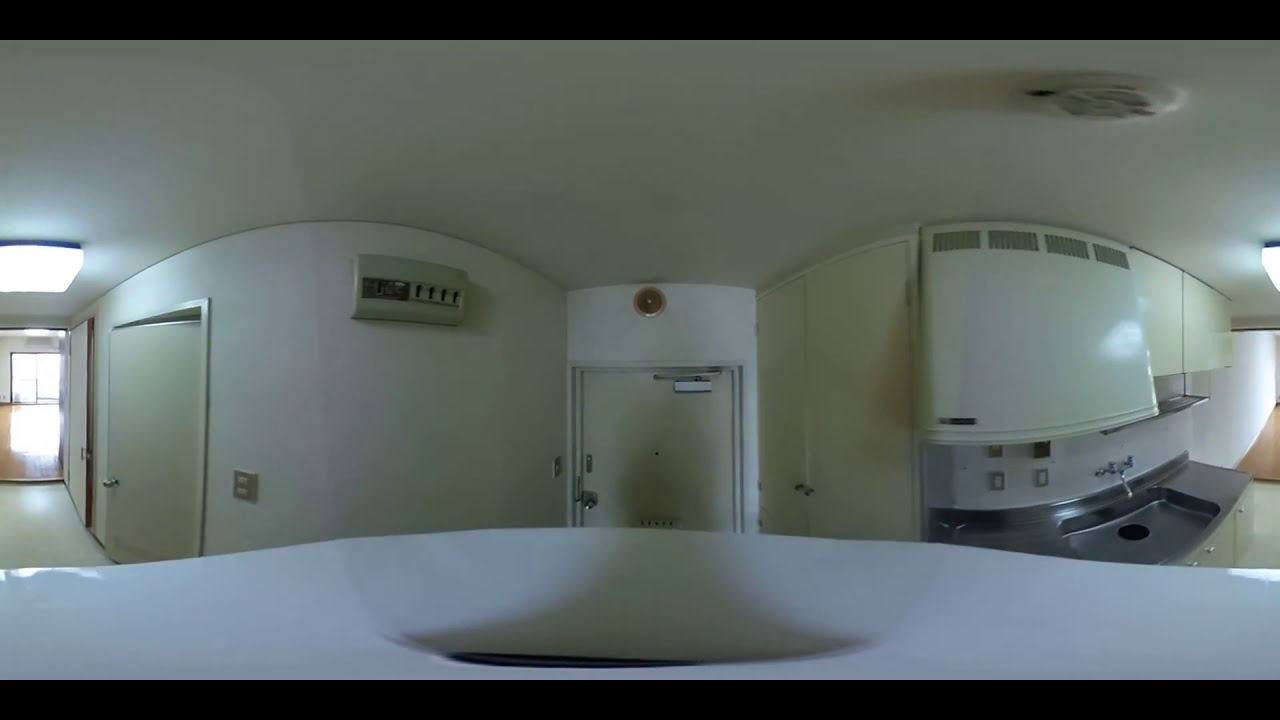The image portrays a wide-angle, panoramic view of what appears to be an apartment interior with the following details:

On the right side is the kitchen area, featuring a gray countertop with a silver sink and a faucet attached to the wall. Above the sink, there's a silver oven hood descending from the ceiling and white cabinets mounted high on the wall. The center of the image is dominated by a beige-colored door, which seems to be the main entrance, next to a beige-colored closet on its right.

Towards the left side of the image, there lies a hallway leading to another door and an opening that reveals a room with brown hardwood flooring. This room, possibly a living room or bedroom, has white walls and a window allowing natural light to enter. The ceiling throughout the main area is white and equipped with a smoke detector. Additionally, there appears to be an air conditioner hanging on one of the walls in the central area.